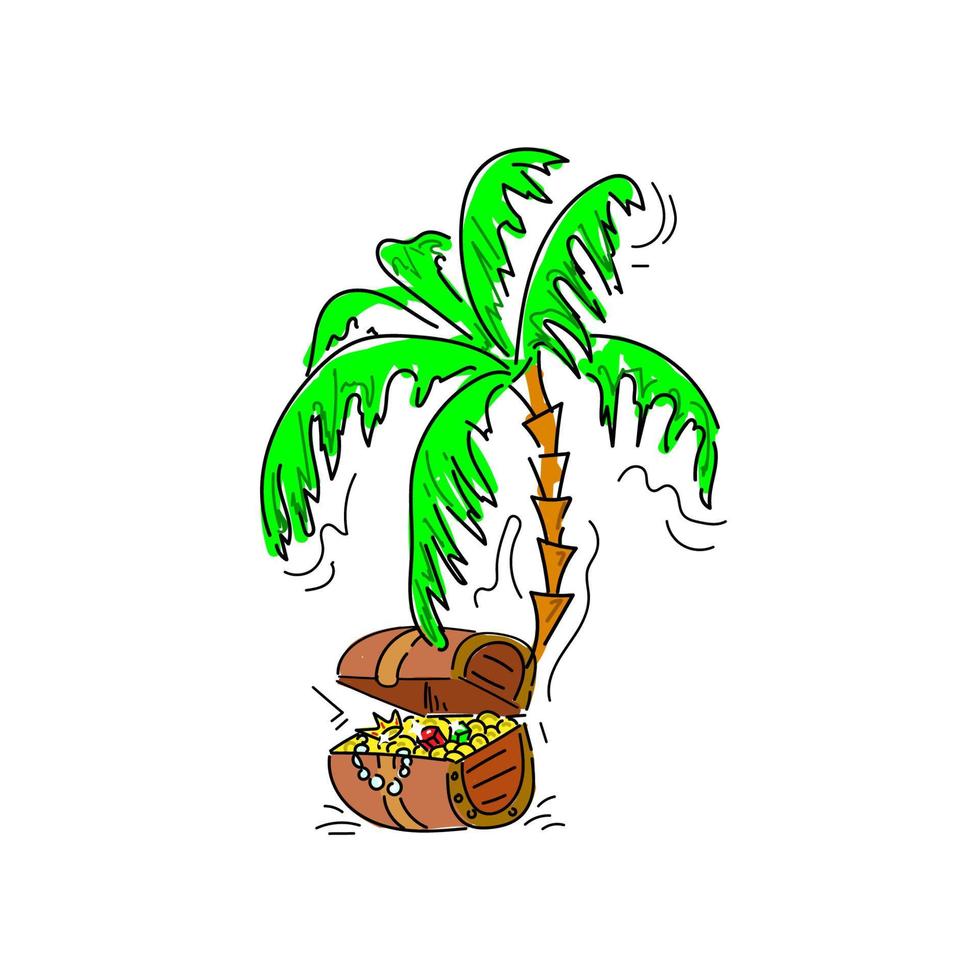In this detailed color illustration, set against a white background, a vividly drawn cartoon palm tree and an overflowing treasure chest are the primary subjects. The palm tree features a light brown trunk made up of stacked, triangular sections outlined in black, curving gracefully to the right before arching back towards the center. Its top is adorned with eight large, bright green fronds, some of which drape over the treasure chest, partially obscuring its open lid. The treasure chest itself is barrel-shaped with a rounded bottom and top, colored in shades of brown and outlined in black. It is brimming with a dazzling assortment of treasures: shimmering gold coins, a delicate pearl necklace, multicolored gems including a ruby, a green cube-shaped gem, and a crown. Black lines around the chest and tree suggest motion, enhancing the dynamic and lively feel of the scene. The overall style is a playful, vibrant cartoon, where the colors overflow slightly outside their outlines, contributing to its whimsical charm.